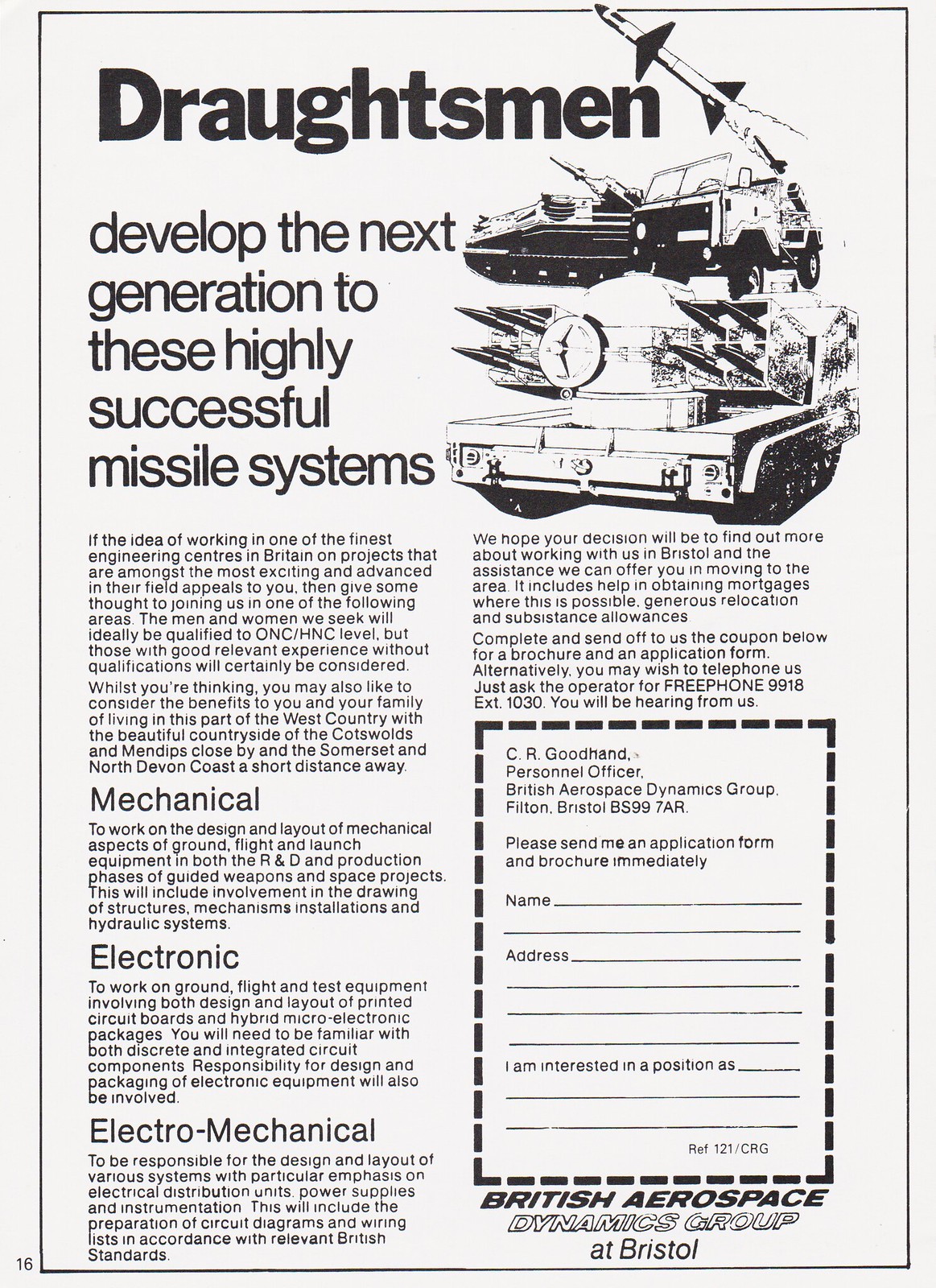The image showcases an aged advertisement, likely pulled from an old magazine, with an off-white, aged-looking background and bold black text. The ad prominently seeks "Draftsmen" to develop the next generation of highly successful missile systems. Positioned in the upper right corner are detailed images of military vehicles, including tanks and missile systems actively launching rockets. The text elaborates on exciting and advanced projects in Britain's finest engineering centers, inviting potential applicants to consider joining in areas of mechanical, electronic, and electro-mechanical engineering.

In the bottom right corner, the advertisement features a form with a dotted line for clipping. This form is addressed to CR Goodhand, Personnel Officer at British Aerospace Dynamics Group, Filton, Bristol BS 997 AR, and requests applicants to fill in their name, address, and their interest in a specific position. The form also prompts for an application form and brochure to be sent immediately. Additional information at the bottom reiterates the British Aerospace Dynamics Group located in Bristol. The entire layout and design indicate an earnest call for skilled engineers ready to work on prestigious and advanced missile systems in Britain.